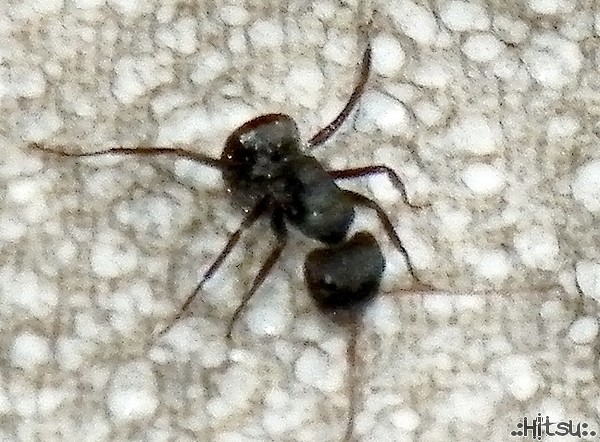This close-up, slightly blurry photograph captures an ant in striking detail against a textured background. The main subject, a six-legged ant with a cylindrical, skinny body and a rounded end, is centrally positioned. The ant's head is round with distinctly long antennae. The insect appears to be very dark brown, almost black, with some hints of lighter brown. It rests on a surface resembling fabric or pebbled paper, exhibiting colors in white, tan, and brown. The background adds to the intricacy with visible fibrous textures. Notably, the word "Hitsu" is featured in small text at the bottom right corner of the image, with three dots on either side, suggesting the name of the photographer. The overall setting of the photo, portrayed in a natural and detailed manner, suggests it might have been taken in a scientific context outdoors, under natural daylight.